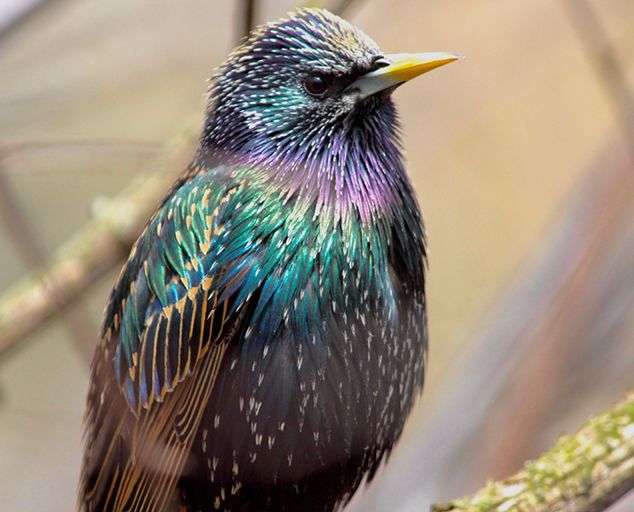In this sharp, nature-photographed image, we see a vibrant, colorful bird perched on a branch in a blurred, cream and light brown background. The bird faces to the right, showcasing its striking yellow and white pointed beak aimed slightly upward. Its head features vivid violet feathers transitioning to a battel color between its black eyes and a lighter purple hue down its neck. Below the head, there's a bright turquoise patch that melds into the bird's chest, adorned with delicate brown feathers accented by white dots. The bird's wings, hanging straight down, exhibit a mix of brown feathers intricately patterned with black lines. The breast area displays a gradient of colors from a deeper purple to green and then black. The branch it perches on, visible in the bottom right corner, is a light wood color accented with green moss. The background remains out of focus but hints at light brown branches and a creamy expanse adding depth to the image. The overall photograph is a testament to the bird's dazzling array of colors and the skillful eye of a nature photographer.